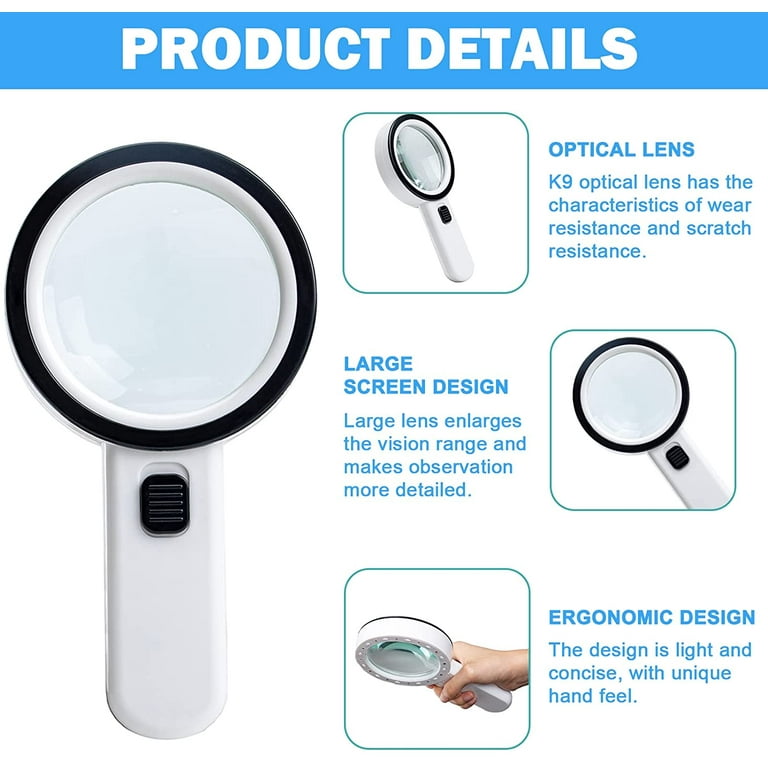This image showcases a computer-rendered online advertisement for a magnifying glass, set against a completely white background. A blue rectangular box with plain white font at the top reads "Product Details." Below this, the left side features a prominent image of the magnifying glass, characterized by its circular lens enclosed in a black rim and a thick white handle equipped with an on-off switch for lighting. The right side of the advertisement presents three smaller images and corresponding feature descriptions in blue font. The first feature, "Optical Lens," highlights the K9 optical lens renowned for its wear and scratch resistance. The second feature, "Large Screen Design," emphasizes a large lens that broadens the vision range for more detailed observation. The third feature, "Ergonomic Design," explains that the magnifying glass is lightweight and concise, offering a unique and comfortable hand feel.